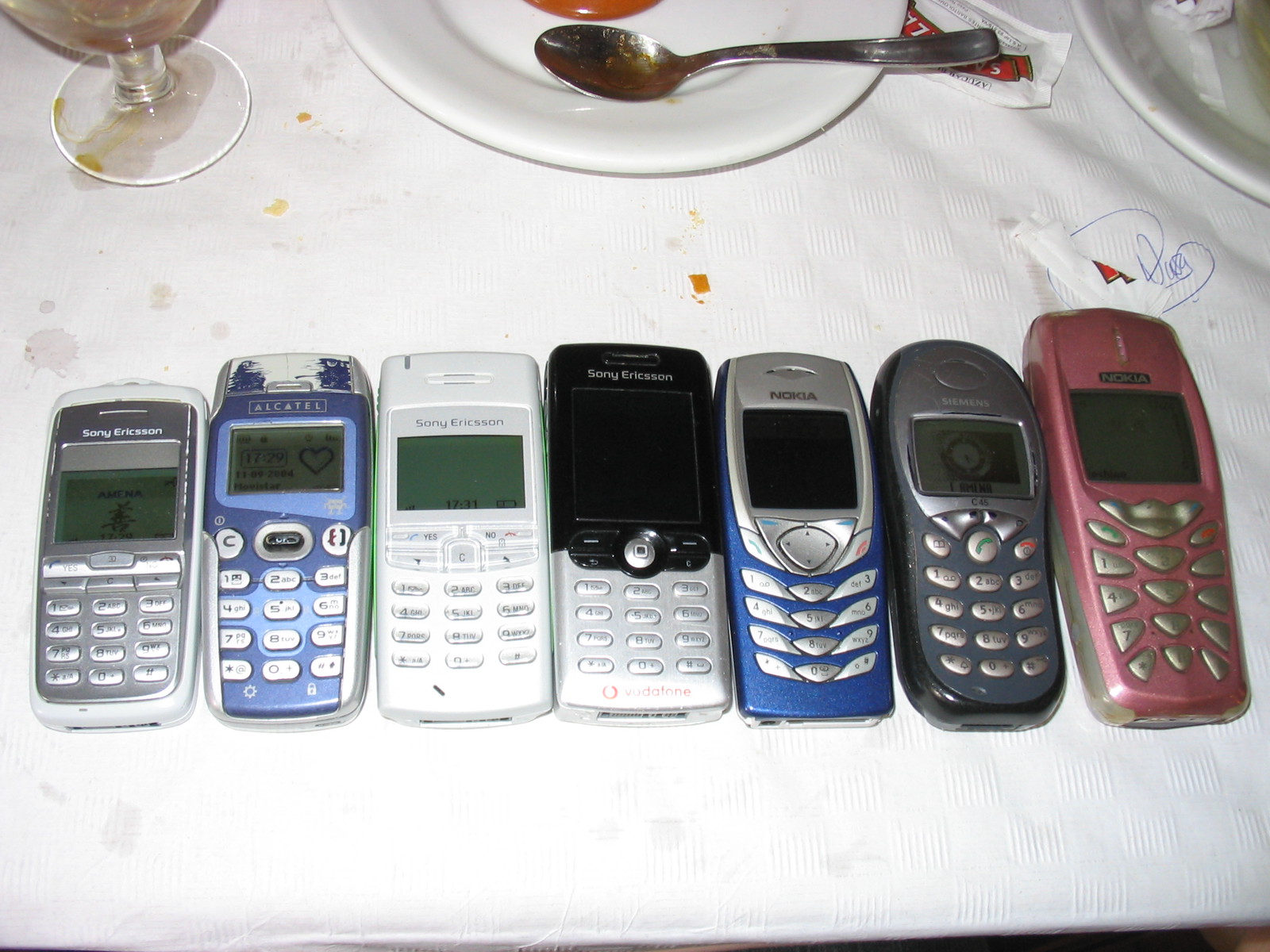This photograph captures an overhead view of a white linen tablecloth, which is marred by food and drink stains, crumbs, and a blue ink signature. The tablecloth features a disorganized scene with seven old-style mobile phones lined up in front of an assortment of dining items. 

In the upper left of the image, a clear glass goblet leaves a stain on the cloth below. Just below it, towards the middle of the photograph, rests a white plate holding a dirty silver spoon tainted with a red sauce, likely ketchup, with an opened condiment packet partly visible beneath the plate. Another plate occupies the upper right corner, featuring a partially seen rolled-up wrapper.

The row of seven vintage mobile phones spans from left to right across the lower portion of the image. The first phone on the far left is a white Sony Ericsson, which is powered on, displaying what seems to be a game. Next to it is a light blue Alcatel phone, visibly worn with its blue exterior faded to white in parts. The third phone is another Sony Ericsson, predominantly white with clearish white buttons and showing the time, 17:31, on its small screen. Following this is a fourth Sony Ericsson, characterized by its black upper half and white number pad. The fifth phone is a Nokia, distinguished by its dark blue body and silver upper half. The sixth phone, marked as a Siemens, features black casing and silver buttons. Finally, the seventh phone is a Nokia, colored in metallic red with silver buttons.

Together, these elements form a nostalgic tableau of outdated technology juxtaposed against the remnants of a messy meal.